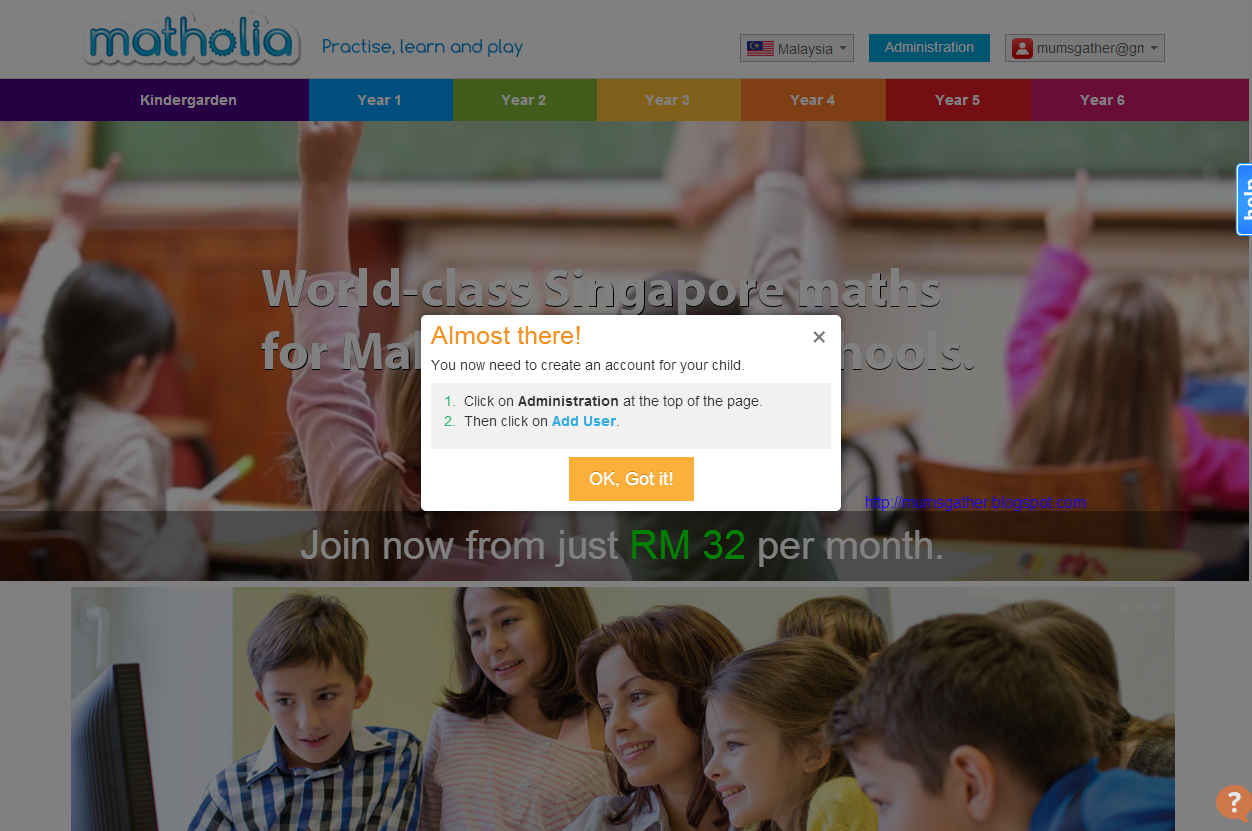The image features a user interface with a gray overlay. At the top, it prominently displays the words "Matholia: Practice, Learn, and Play,” accompanied by a small Malaysian flag and a downward arrow. Directly below, a blue box with "Administration" indicates the administrative section. Adjacent to it, there is an icon with a red figure and some text that is illegible. 

The middle portion of the image presents a colorful layout categorizing various educational levels: "Kindergarten" in purple, "Year 1" in blue, "Year 2" in green, "Year 3" in yellow, "Year 4" in orange, "Year 5" in red, and "Year 6" in purple. Each category is associated with pictures of children and the phrase "World-Class Singapore Maths."

Towards the bottom section, a large white box contains the message, "Almost there, you now need to create an account for your child," with an "X" in the corner to close the box. Instructions follow in a blue box: "1. Click on Administration at the top of the page," and then "2. Click on Add User," accompanied by an orange button that reads "Okay, got it." Below this, there's a call-to-action text, "Join now from just RM 32 per month."

In the corner of the image, there is a picture of a teacher surrounded by children, emphasizing a collaborative learning environment. Finally, on the bottom right corner, there's a small orange circle with a white question mark, presumably an icon for help or more information.